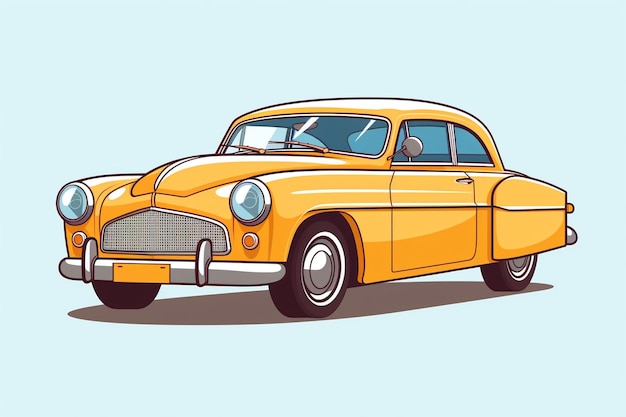This detailed, color illustration showcases a pristine yellow two-door vehicle, likely hailing from the mid to late 1950s. The car is depicted at a diagonal angle, highlighting its front end where classic round headlights are framed by a gleaming metal grille. The vehicle's exterior boasts a lustrous finish, reflecting light to accentuate its vintage charm. It rolls on black tires featuring polished silver hubcaps. Clear details include windshield wipers positioned to the left and a rearview mirror mounted on the driver's side. The car casts a realistic shadow beneath it, enhancing the depth of the illustration. Set against a solid light blue background free of any text, people, plants, animals, or buildings, the image draws complete focus to the timeless elegance of this mid-century automobile.